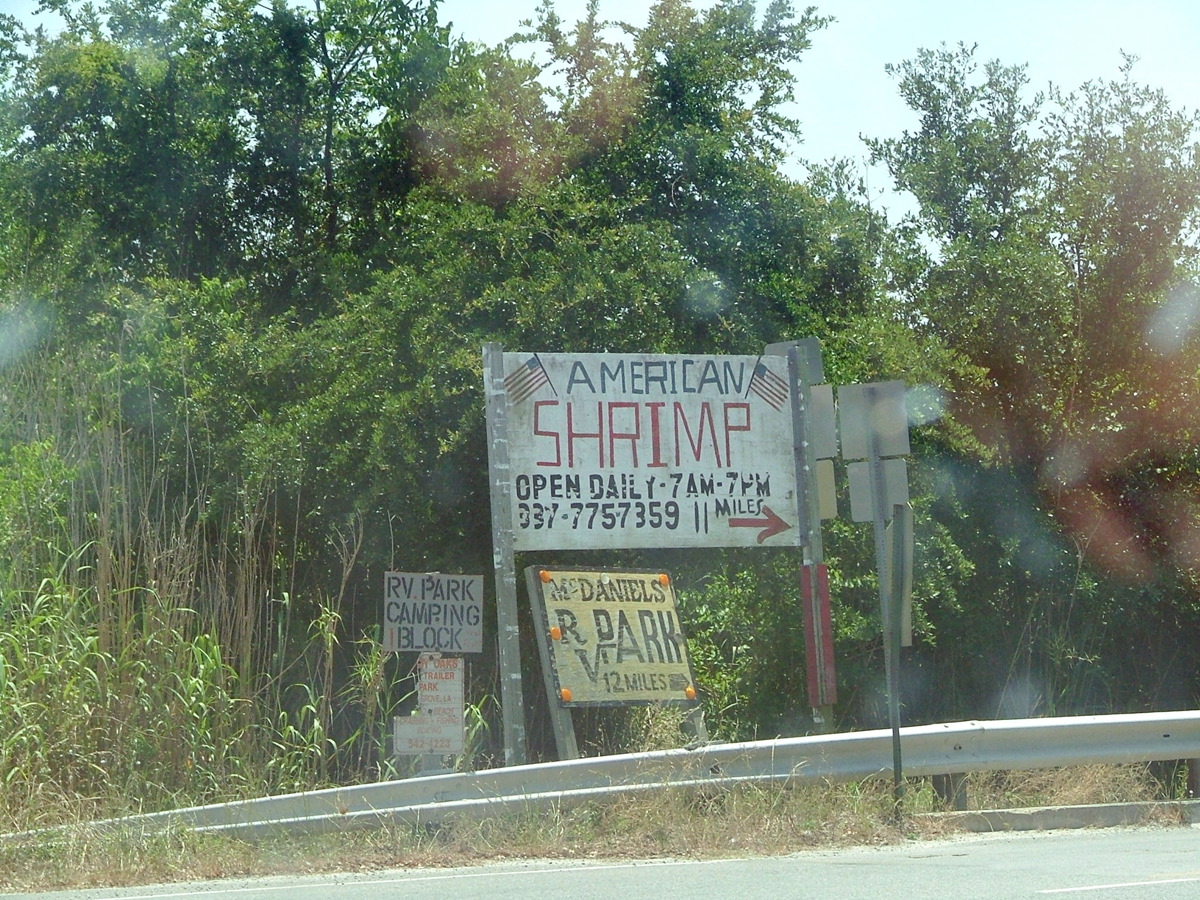This photograph depicts a collage of handmade signs situated along the side of a road, bordered by a silver guardrail. The focal point is a tall wooden post showcasing the largest sign. This sign reads "American Shrimp," with "American" in blue and "Shrimp" in larger, bold red letters. Flanked by two American flags, it boldly announces: "Open Daily 7 a.m. - 7 p.m." Below, additional text provides the distance: "11 miles" with a red arrow pointing to the right.

Beneath the primary sign is another that advertises "Miss Daniels RV Park," indicating it is 12 miles away, also to the right. This sign features a yellow background with black text. There is also another nearby sign offering "RV Parking & Camping Block" instructions.

The signs are positioned near the edge of a road, with a variety of trees and bushes providing a natural backdrop. The scene is set under a clear blue sky, enhancing the vividness of the image. The brown grasses visible in front of the guardrail emphasize the rustic setting.